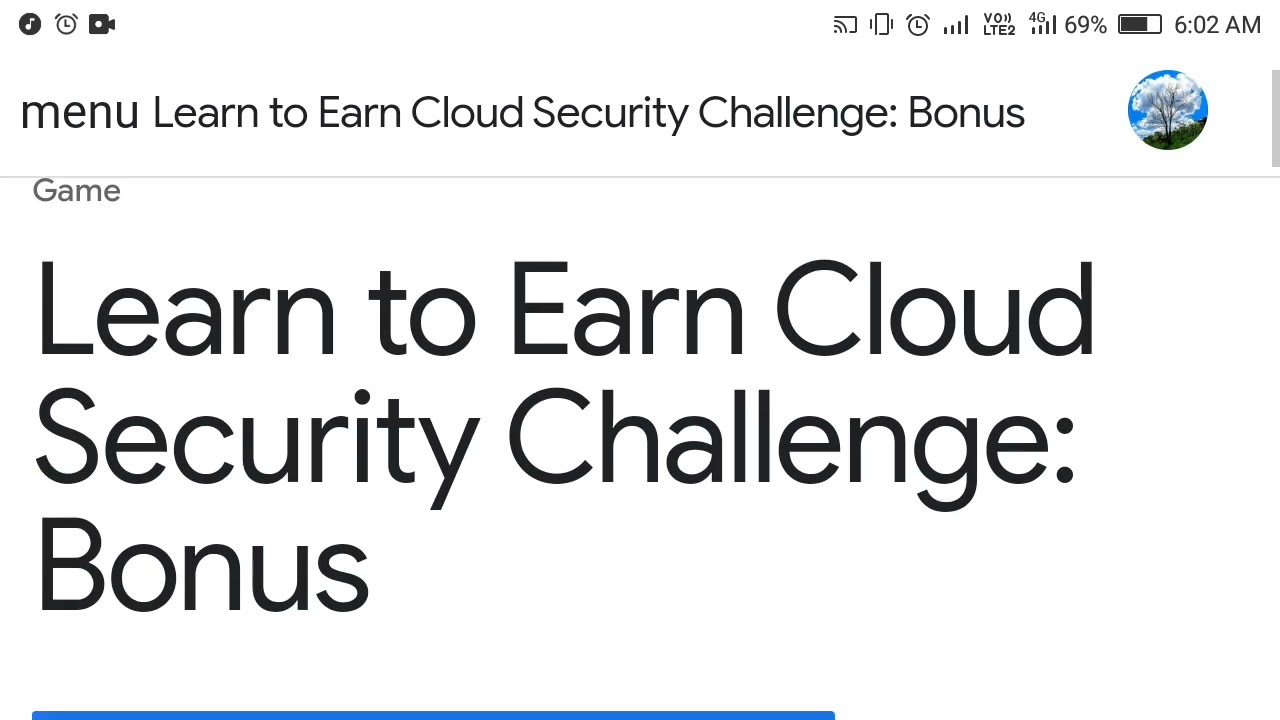This image is a detailed screenshot from a digital device, either a laptop, cell phone, or tablet, in a landscape orientation. At the very top of the screen, against a white background, various icons are visible including an alarm, a video camera, and a clock on the upper left, with the time reading 6:02 AM and a battery indicator at 69% on the upper right. Below these icons, the header features black text that reads, "MENU Learn to Earn Cloud Security Challenge Bonus," accompanied by a circular logo to the right depicting a tree against a sky-blue background on a green hill. Further down, also against the white background, larger bolded black text repeats, "Learn to Earn Cloud Security Challenge Bonus." A thin blue horizontal line runs below this text, stretching across two-thirds of the screen.